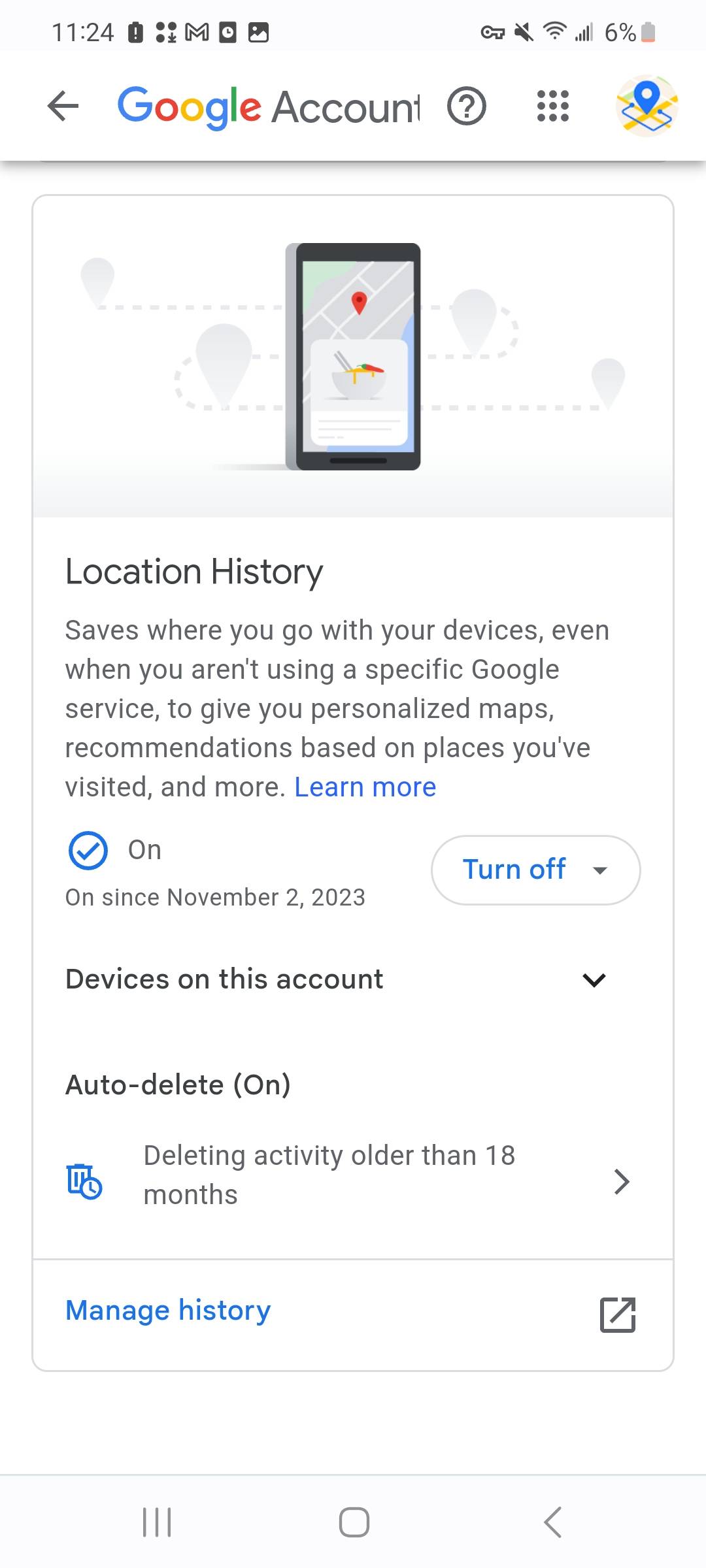**Descriptive Caption:**

The screenshot displays a mobile phone interface set against a completely white background. At the bottom row, three distinct icons are present: the first icon features three vertical lines side by side, the middle icon is a square, and the last icon is a triangle pointing towards the left.

At the top banner, the left-hand corner shows the time "11:24". Moving right, there's a battery icon followed by a sequence of symbols — a cluster of four small squares, three additional squares paired with a star, a letter "M", a clock icon, and an icon indicating an image. On the far right of the top banner, additional icons are visible, including a key, a speaker with a line through it (indicating mute), the Wi-Fi signal, cellular signal strength, a battery percentage showing "6%", and a battery icon indicating a red sliver, denoting low battery life.

Below this top banner sits a gray arrow pointing left, adjacent to the text "Google Account". Following this, there’s a gray ring encircling a white circle with a gray question mark in the center. Next to this is an icon resembling a stack of circles organized in three rows of three. On the far right, an icon depicts a map with a blue location marker.

The main window open on the screen is titled "Location History". It features an illustrative graphic showing location tags connected by dotted lines, a cartoon image of a mobile phone displaying a map, and a bowl of ramen with an orange location tag. Below the image, the text explains, "Location History saves where you go with your devices, even when you aren’t using a specific Google service, to give you personalized maps, recommendations based on places you’ve visited, and more. Learn more."

Directly beneath this explanation, a blue ring encircles a white circle with a blue checkmark in the center, accompanied by the text "On, On since November 2nd, 2023." To the right is a tab labeled "Turn off" with a down arrow, which remains unselected. Further options include "Devices on this account" with a down arrow for expanding the view, "Auto-delete (On), Deleting activity older than 18 months" illustrated by a trash can and clock icon with a left-pointing arrow, and "Manage History" alongside a square icon with an upward-diagonal arrow.